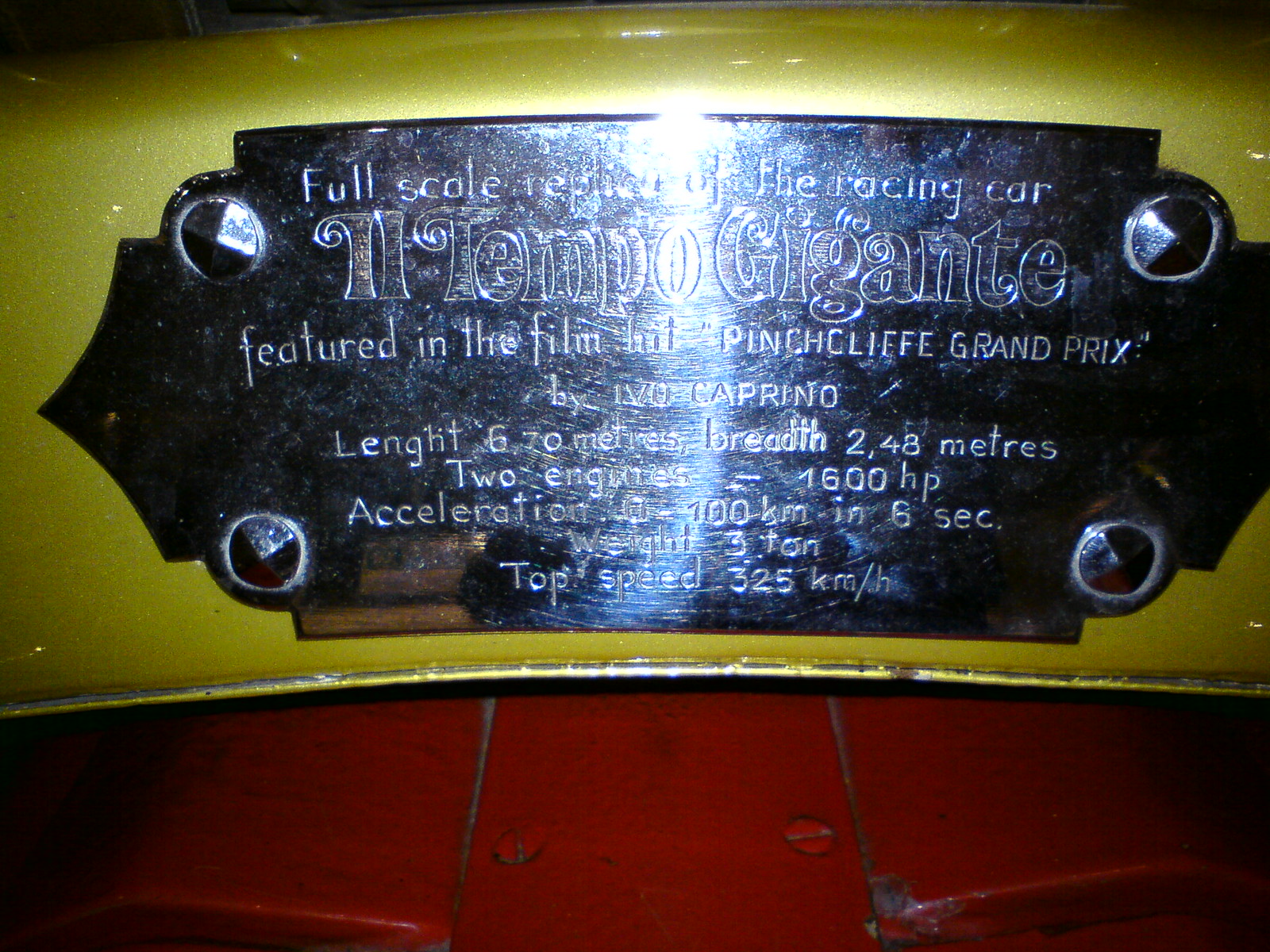The image depicts a detailed metallic plaque mounted on a vehicle. The top portion of the background is a shiny yellow metal, transitioning to a red metal piece at the bottom. This smooth metallic surface has a polished, reflective quality that creates glare, making parts of the plaque difficult to read. The plaque itself is dark brown or black, secured by four bolts. The text on the plaque reads:

"Full-scale replica of the racing car Tempo Gigante, featured in the film Pinch Cliff Grand Prix by Ivo Caprino. Length: 6.70 meters, Breadth: 2.48 meters, Two engines: 1,600 horsepower, Acceleration: 0 to 100 kilometers in six seconds, Weight: three tons, Top speed: 325 kilometers per hour."

This plaque is attached to the front of the vehicle and serves as an explanatory label for its specifications and origin.